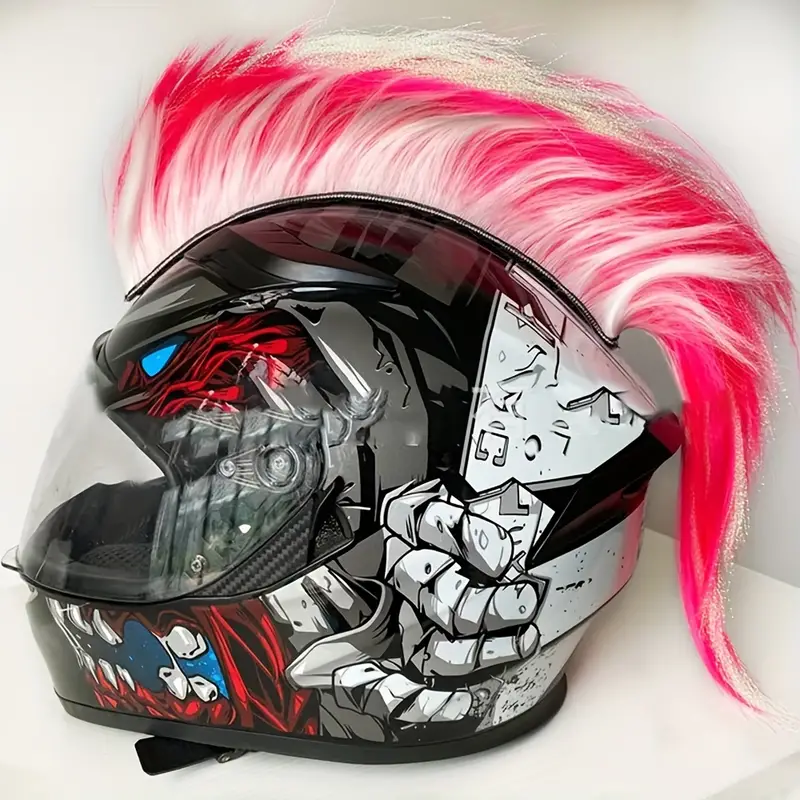The image depicts a striking custom motorcycle helmet facing left, predominantly black with an array of meticulous designs. Topping the helmet is a distinctive mohawk composed of vibrant red and white hair, trailing neatly to the back of the helmet. The mohawk is centrally positioned, adding a wild and unique flair. 

The side and front surfaces of the helmet feature complex, metallic-themed artwork. On the right side, there's a detailed depiction of a hand prying at what appears to be metallic sections, painted in a gray and white color scheme. The left side showcases a sinister, zombie-like mouth with exposed muscles, saliva, and teeth, some of which are missing, revealing a blue night sky pattern behind them.

Above the artwork is a transparent fishbowl visor through which the helmet's black cushioned interior is visible, including where the wearer’s eyes would be. The visor is clean and offers full visibility. Adding to the intricate details, there are menacing blue eyes depicted on the top of the helmet amidst a muscly texture design.

The helmet rests securely on a white table against a white background, with a buckle visible underneath, ready for fastening. Overall, this exceptional piece combines artistry and functionality, making it a standout accessory for any motorcyclist.